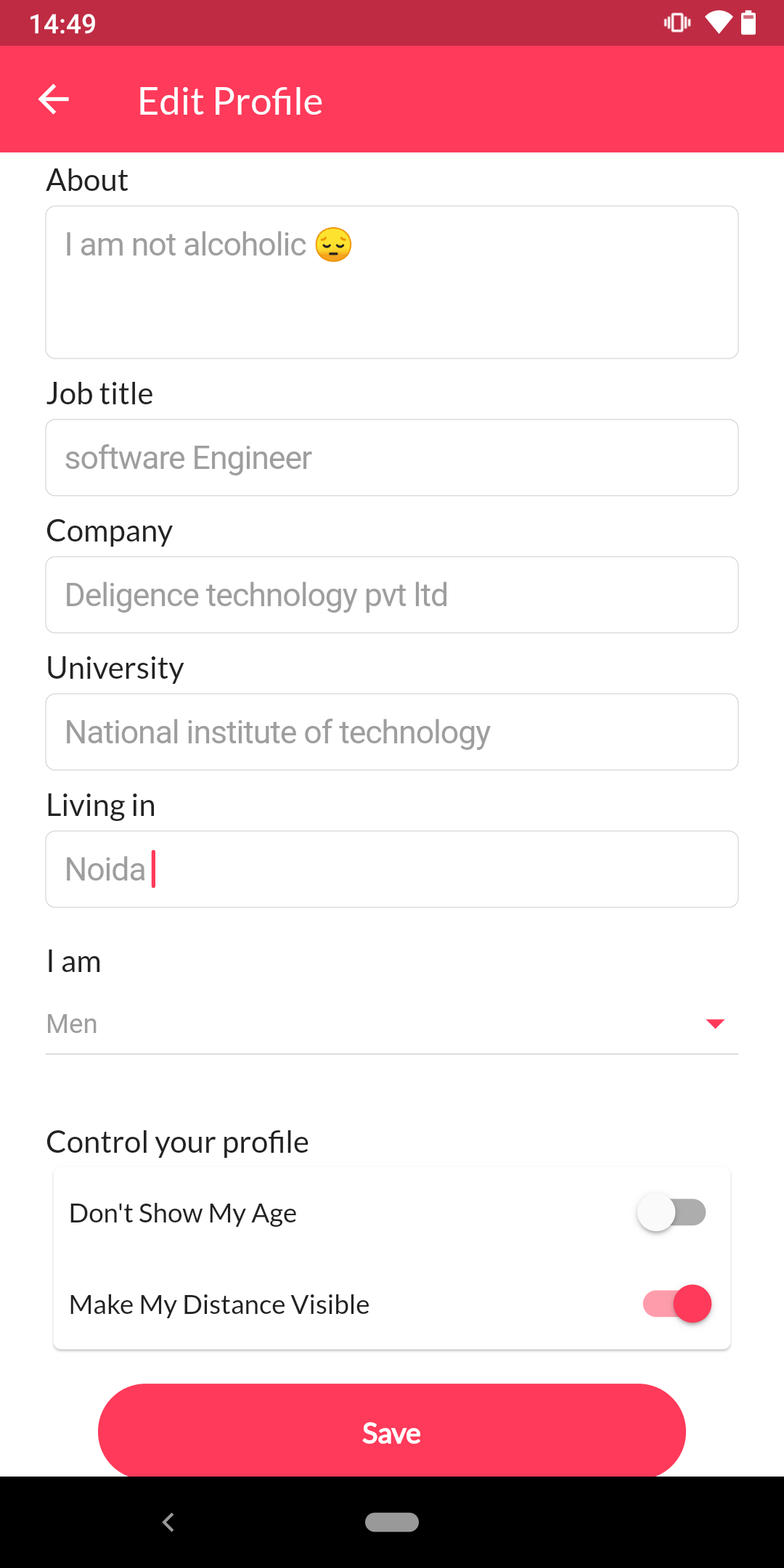A detailed screen capture from a cell phone displaying a user filling out an "About Me" page on an application. The image is dominated by a two-tone red banner at the top: a deep crimson border on the very top, just shy of brown, followed by a vivid red section below it. All text, icons, and symbols in this red area are white, providing a stark contrast. 

In the top left corner, the time is shown as 14:49. On the top right, three icons are displayed sequentially: a cell phone symbol, a triangular Wi-Fi symbol, and a nearly full battery icon. Below this, in the solid red section, there's a left arrow and the words "Edit Profile."

The main content begins with a label titled "About" in black. The corresponding text box beneath it contains the phrase "I am NOT an alcoholic" followed by a looking-down emoji. Below this, the next labeled field is "Job Title" with "Software Engineer" filled in the text box. Following that is the "Company" label, with "Diligence Technology Private Limited" entered. The subsequent field is "University," filled with "National Institute of Technology." In the "Living In" section, "NOIDA" is specified.

The final input section includes "I am" with "Men" selected, indicated by a red dropdown arrow on the right. Further control options for the profile are displayed in black text on a white background: "Don't Show My Age" is turned off, and "Make My Distance Visible" is turned on. A rectangular red button labeled "Save" in white is prominently placed for saving the changes. At the very bottom, a black bar with a back left arrow offers an option to return to the previous screen.